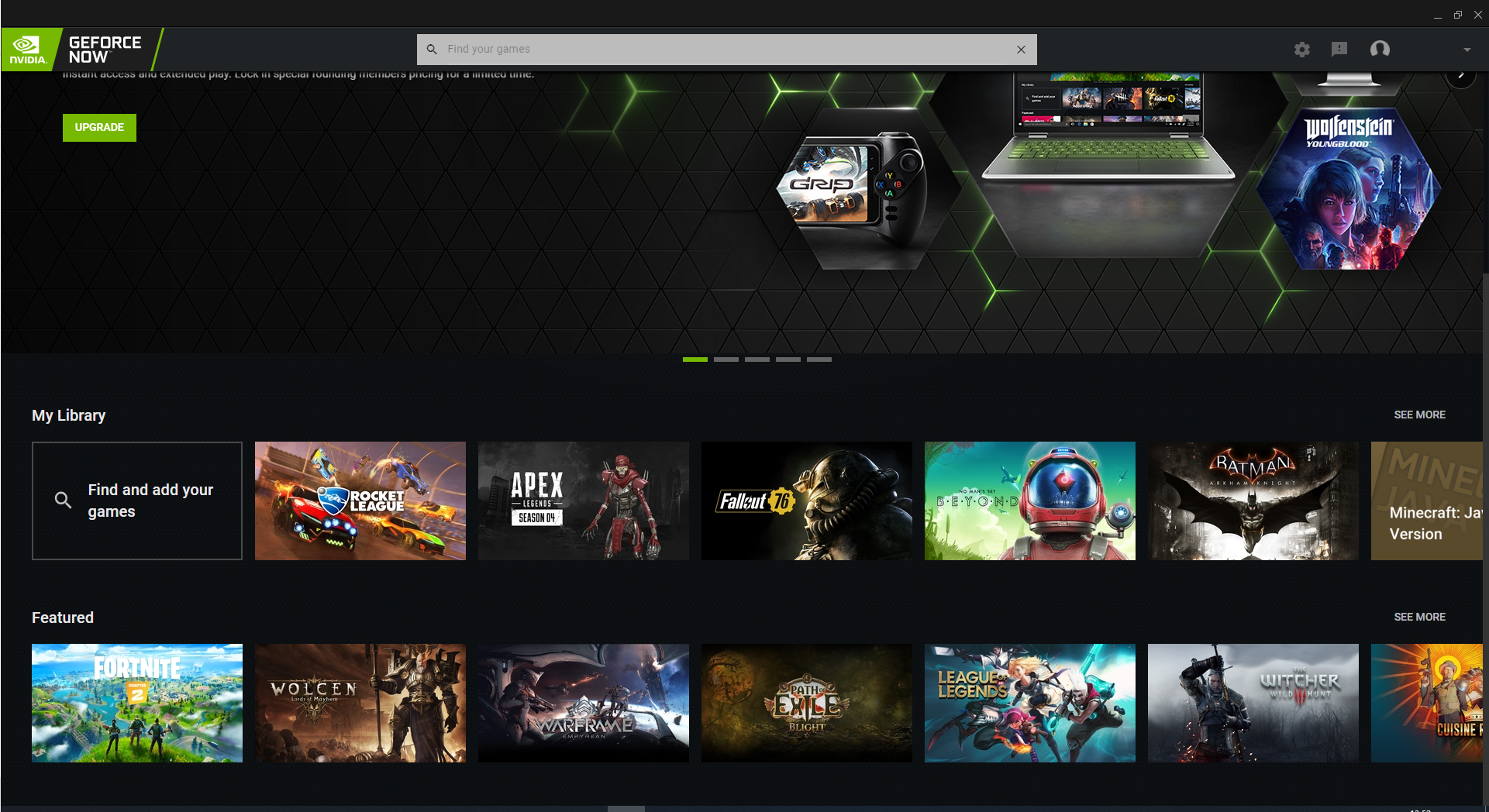**Caption:**

A screenshot of the NVIDIA GeForce Now promotional interface. At the top left corner, the iconic NVIDIA logo is presented inside a green box with the text "NVIDIA" in white. Adjacent to it is the GeForce Now branding. The promotional message reads, "Instant access and extended play. Lock in special founding members pricing for a limited time." 

A search bar labeled "Find your games" is located centrally, accompanied by a green rectangle button labeled "Upgrade" in white letters. To the right, an image of a gaming laptop rests on a steel cube, emphasizing the platform’s multi-device compatibility. Adjacent to it on the left side, there is an image of a handheld gaming device.

To the right, an octagonal badge displays the title "Wolfenstein: Youngblood." The bottom section transitions into a list titled "My Library," showcasing various games such as Rocket League, Apex Legends Season 4, Fallout 76, No Man's Sky Beyond, Batman Arkham Knight, and Minecraft Java Version.

Further down, a "Featured" section highlights popular games including Fortnite, WOLCEN, Warframe, Path of Exile: Blight, League of Legends, Witcher 3: Wild Hunt, and another game partially cut off at the image's right edge.